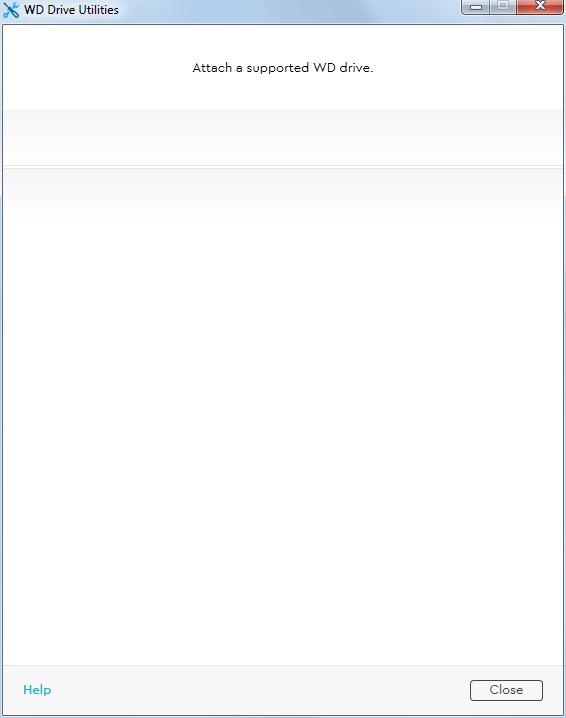In the image, we observe an interface that appears to be the main screen of a web or application page, designated for WD Drive Utilities. At the top left corner, there's a logo composed of a dark blue screwdriver and a light blue wrench crossed to form an 'X' shape. Beside the logo, the text "WD Drive Utilities" is displayed.

On the top right corner, there are three interactive icons for window management: Minimize Screen, Maximize Screen, and Close Screen. Below this header, there is a message highlighted in a white font against a black background, prompting the user to "Attach a Supported WD Drive."

The central portion of the interface is predominantly blank, featuring a light gray header box followed by a subtle double line separator of the same color, which accentuates the emptiness of the overall area. 

At the bottom left corner, there is a blue "Help" button for user assistance. On the opposite side, at the bottom right corner, a square button labeled "Close" is present, presumably to exit the application or window. The general aesthetic is minimalistic, providing essential information and navigation options without clutter.